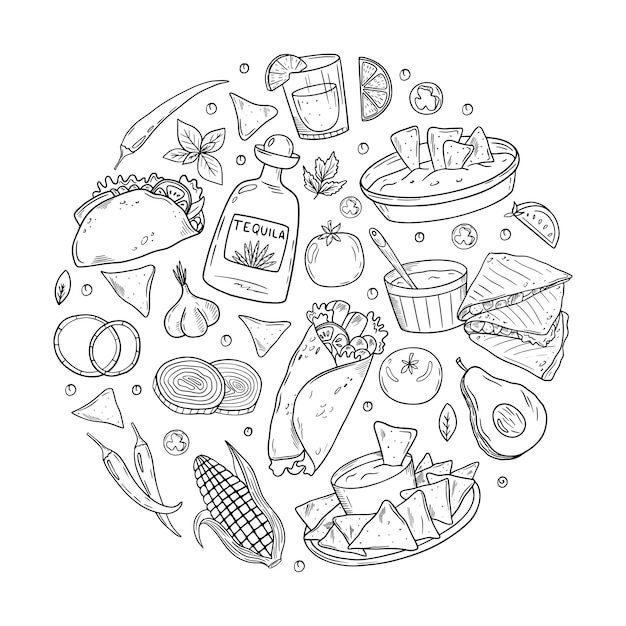This black and white graphic image presents a circular arrangement of various Mexican cuisine items against a white background. At its center, prominent items include a bottle of tequila and popular foods such as tacos, tortilla chips with dips likely to be salsa or guacamole, and an ear of corn. Surrounding these are numerous smaller elements including an avocado, onions, garlic, cilantro leaves, tomatoes, a lime wedge, and hot peppers. The circle is densely packed with these items, creating a rich depiction of Mexican cultural foods and drinks, accentuated by fine details such as a glass with a lime slice, vegetable slices, and even small beans. The intricate design showcases around 30 objects, all contributing to a vibrant representation of the cuisine.